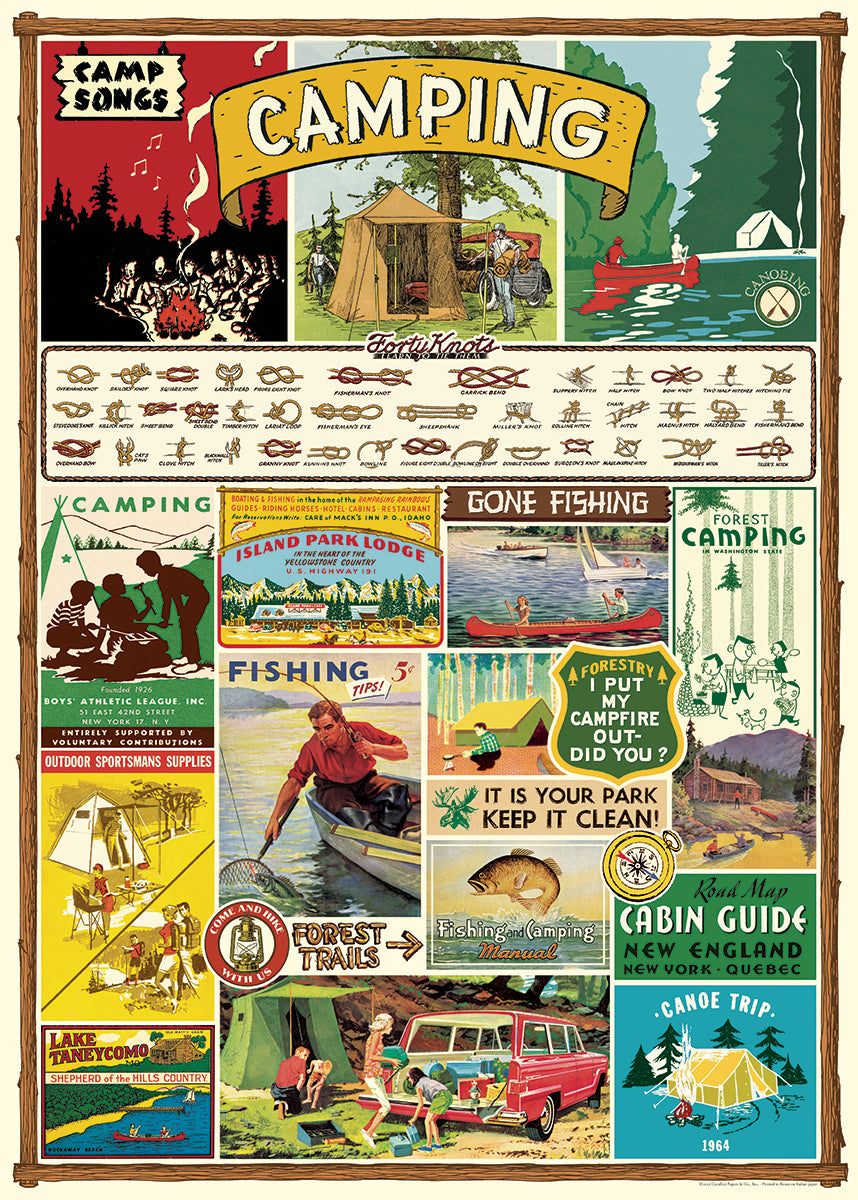The image appears to be an illustration from a camping guide or magazine, designed with a rustic, wood-like border that frames the vertically oriented, rectangular poster. At the top, a yellow banner prominently features the word "CAMPING" in large, bold white letters. Beneath this banner, there is a collage of three images portraying quintessential camping scenes: campers gathered around a campfire singing songs, a pitched tent, and adventurers canoeing or kayaking. Below these vibrant visuals, the phrase "40 knots" is displayed in cursive, accompanied by meticulously illustrated examples of 40 distinct rope knots—each compact and precisely labeled against a clean white background. The bottom portion transitions into a collection of assorted slogans and miniature advertisements related to camping activities, such as "Gone Fishing," "Fishing Tips," "Forest Trails," "Cabin Guide," and suggestions for various outdoor adventures, including car camping and back-of-the-car setups. The overall design captures the essence of camping, blending practical information with inviting imagery to create an engaging and informative layout.